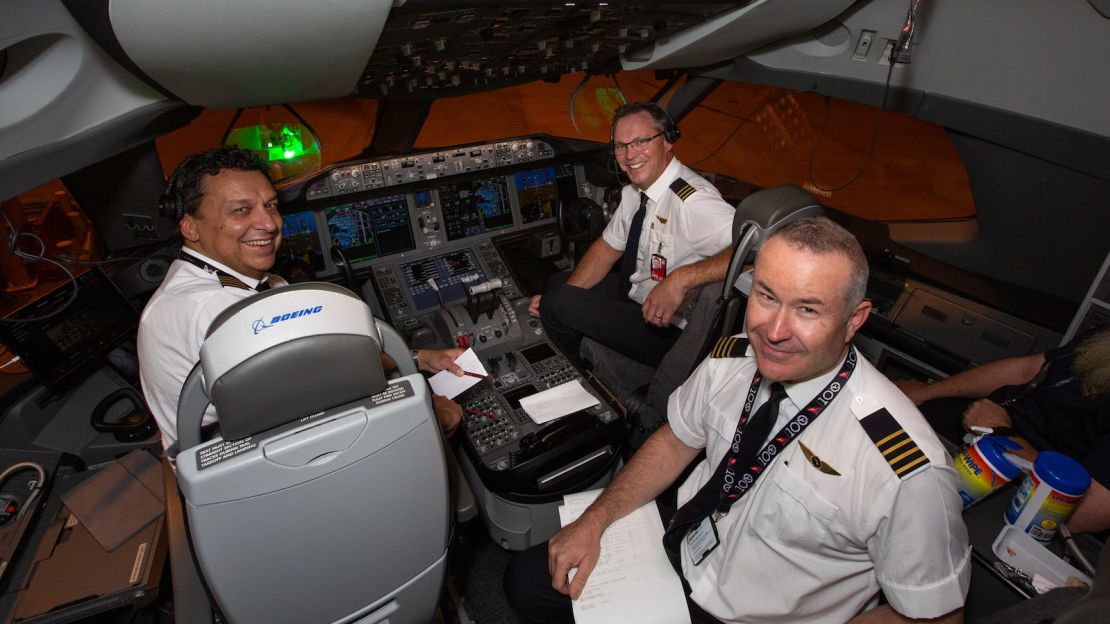The photograph is taken from an overhead perspective, capturing an interior view of a Boeing aircraft cockpit. It features three middle-aged men, all adorned in traditional pilot uniforms with black epaulettes bearing yellow stripes and wings insignia above their chest pockets. Each man is wearing a white shirt with cuffed short sleeves and a black tie. The central figure, positioned directly in the pilot's seat showcasing the Boeing logo, is a slightly brown-skinned man with a broad smile. He is flanked by a Caucasian man on his right, who is distinguished by glasses and a similarly cheerful expression. The third man, standing behind the central console full of complex controls and screens, is also Caucasian, with short graying hair and a lanyard around his neck, holding white papers as if taking notes.

Further emphasizing the camaraderie, all three individuals are seen smiling, perhaps during a training session within what appears to be a simulated cockpit environment. This suggestion is bolstered by the visible orange shield outside the cockpit windows, hinting at a possible training rig. Additional context from the era of COVID is provided by the presence of multiple containers of disinfecting wipes, implying a heightened focus on cleanliness. The setting is intimate, bustling with the sophisticated navigation and control equipment characteristic of a large commercial aircraft such as a Boeing 747 Dreamliner. The atmosphere is further detailed by visible sections of the cockpit walls framing the upper part of the photo, engulfing the trio in their professional environment.